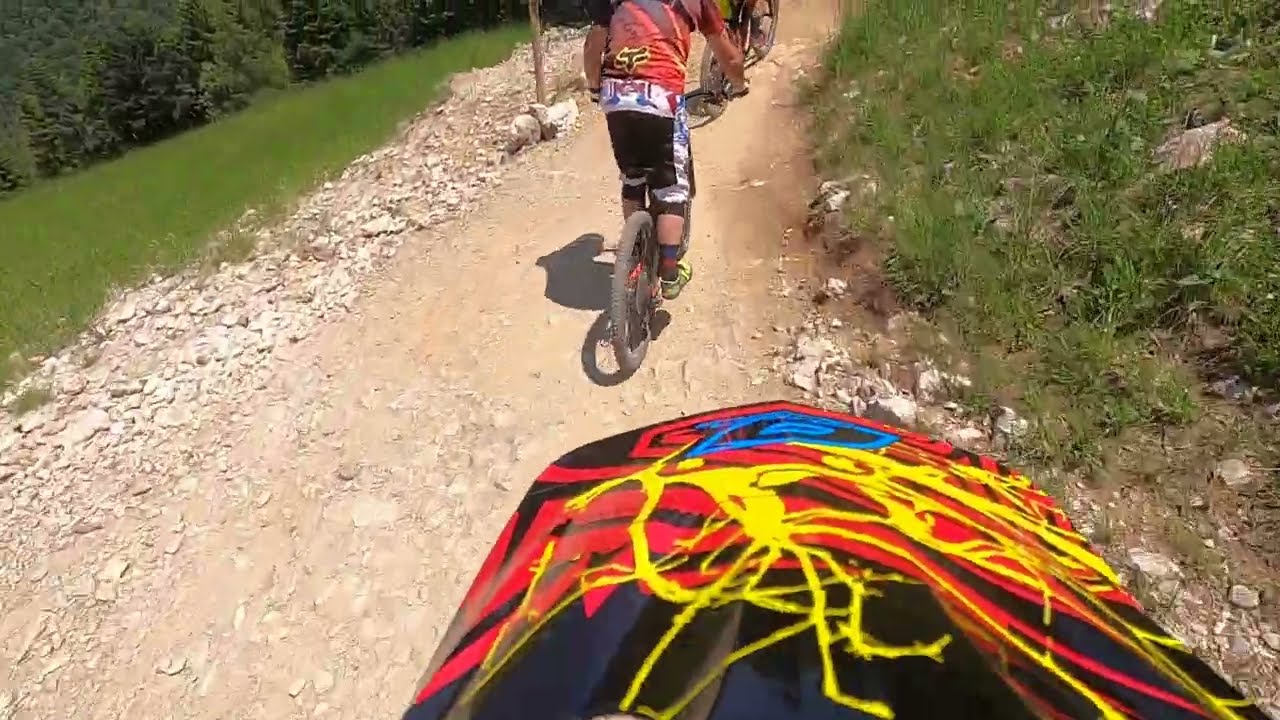In this detailed outdoor scene, we see a dirt and rocky BMX bike trail extending upward through the center of the image. Flanked by grassy hills on both sides, with a noticeable downward slope on the left, the path draws the eye inward. Various riders populate the trail, with two BMX bicycles visible and one rider seemingly taking the photo from their bike. The rider in the middle is distinctively dressed in a red t-shirt with a Fox motocross logo on the back, paired with shorts, yellow sneakers, and black socks. The backdrop showcases a park-like setting with trees, and although the sky is not visible due to the camera angle, the bright lighting suggests it is midday. The image bursts with a vibrant palette of colors: green from the grass and trees, tan and rocky browns of the trail, and the various hues worn by the riders—white, black, yellow, red, blue, and orange. Importantly, there is no visible text in the image, and for more information, one might visit www.FEMA.gov.